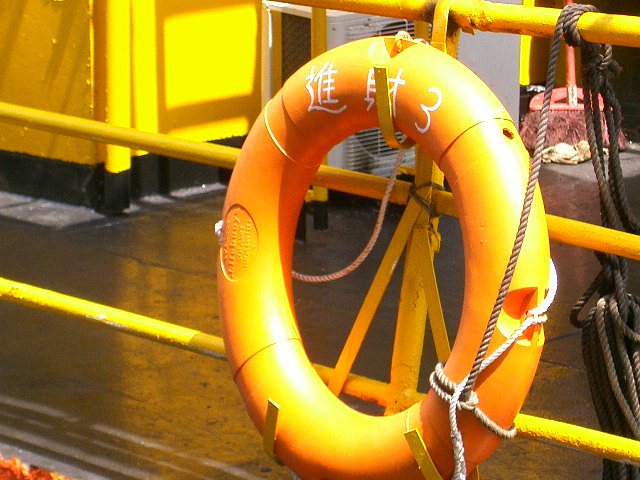The image showcases an orange life preserver hanging prominently on a yellow steel railing aboard a ship. The life preserver is marked with hand-painted, white symbols in what appears to be Chinese or Japanese, and features a number three. Attached to the life preserver is a white rope. The ship's deck is visible, likely composed of black material, with yellow compartments behind the life preserver. Additional elements in the background include white containers and a red broom situated in the top right corner. The entire scene is bathed in sunlight, emphasizing the outdoor setting and the functional maritime environment.